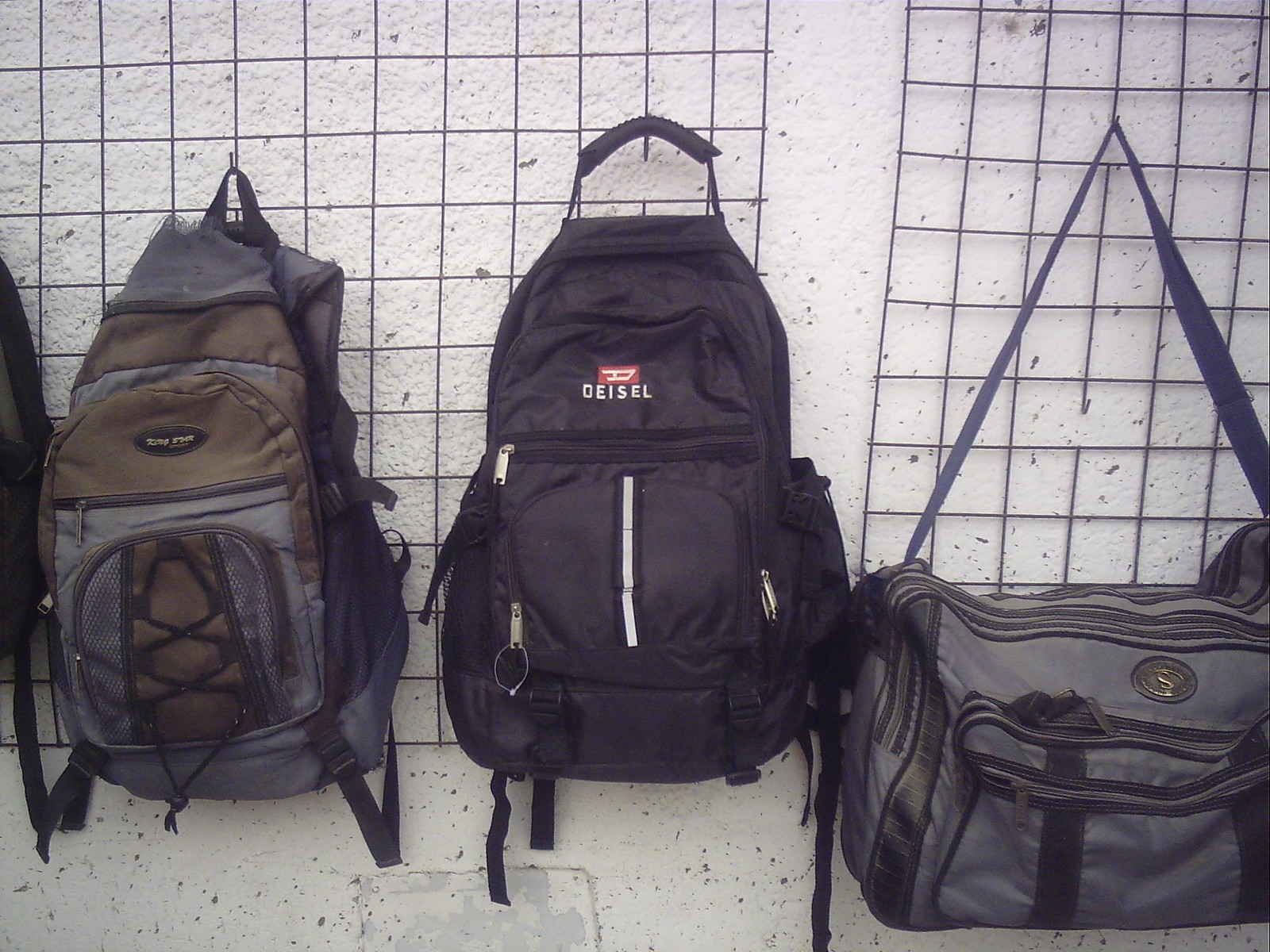The photograph features a display, likely taken in a retail or outdoor market setting, showing a white, pitted stone wall with gray or black speckles, which serves as the backdrop. Suspended from a wire grid or rack mounted on this wall, four bags are presented, though only three are fully visible. 

Starting from the left, the first bag is a hiking-style backpack, primarily in shades of light and dark brown with some gray areas. It shows signs of wear and tear, with a noticeable rip, zip string, and mesh compartment on the front. 

The central bag is a black canvas backpack in relatively good condition. It features silver zippers, a reflective gray stripe, and a prominent red and white "Diesel" logo, suggesting it may be a knockoff of the well-known brand due to the spelling variation in some descriptions.

To the right, the image includes a gray duffel or gym bag, hanging by a longer shoulder strap. This bag has several zippered pockets and compartments, and like the other bags, it shows signs of wear, including a visible rip and a small gold circular emblem on the front.

The photograph also captures just the very edge of another bag on the far left, hinting that there are more bags in this display, aligning with the scene that suggests the bags are likely being sold.